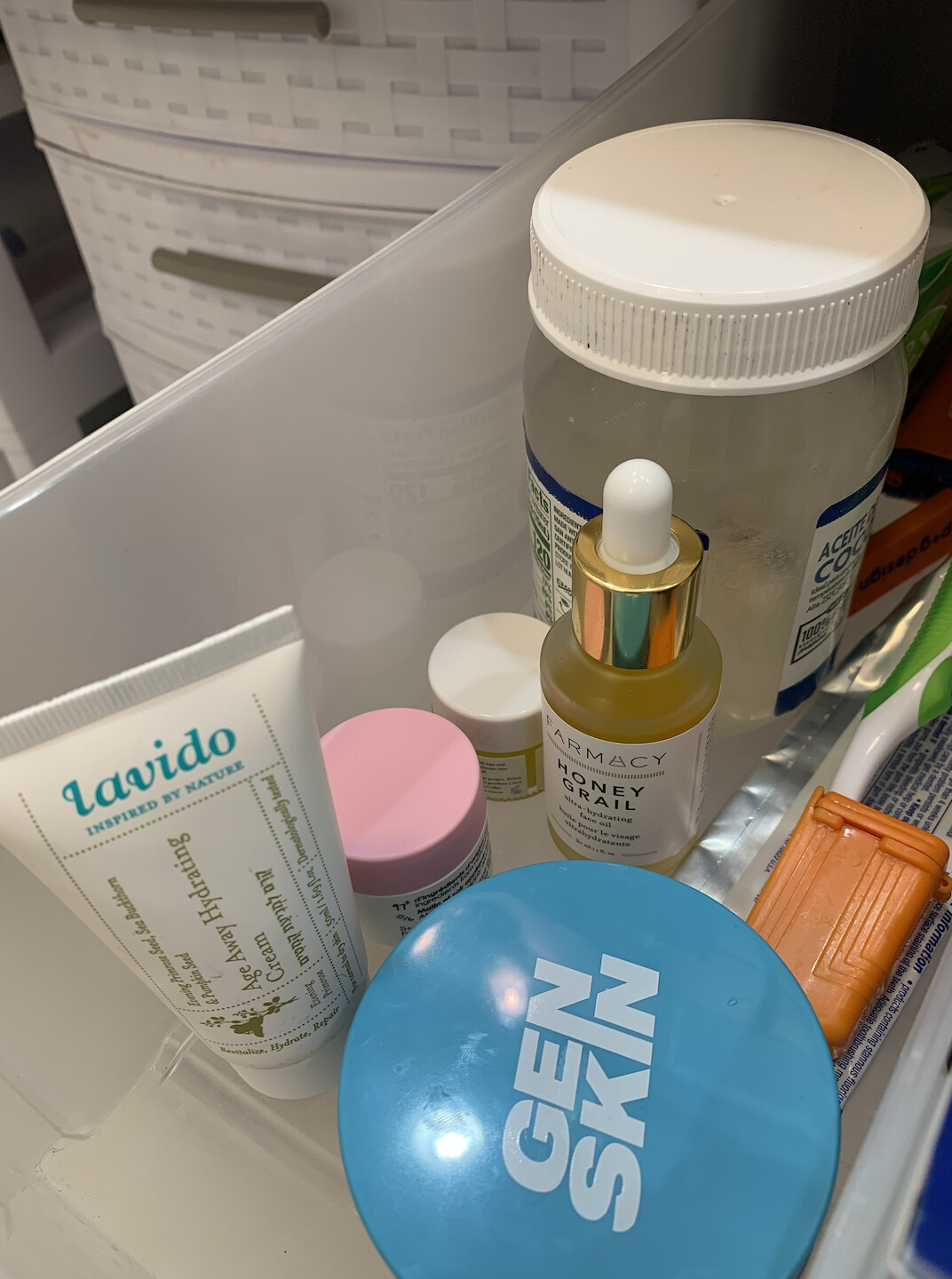The photograph is taken inside a deep plastic bin located in a bathroom. The bin holds various Health and Beauty Aid products, meticulously captured in detail. The first visible item is a container with a blue circular lid and white lettering, labeled "Gen Skin," with "Gen" spelled as G-E-N. Adjacent to it is a squeeze tube with blue lettering, marked "Levito." The small print under "Levito" reads "Inspired by Nature," indicating that it is an age-away hydrating cream.

Further into the bin, there are a couple of small pots with illegible labels. One of the pots has a pink lid, and the other has a white screw lid, possibly containing eye cream. Additionally, there's a dropper bottle labeled "Pharmacy Honey Grail," which is a golden-colored substance, likely an oil or serum. 

Finally, a toothbrush with a white plastic handle and green accents is also visible at the edge of the bin. The well-organized assortment of beauty products suggests a focus on skincare and personal care.